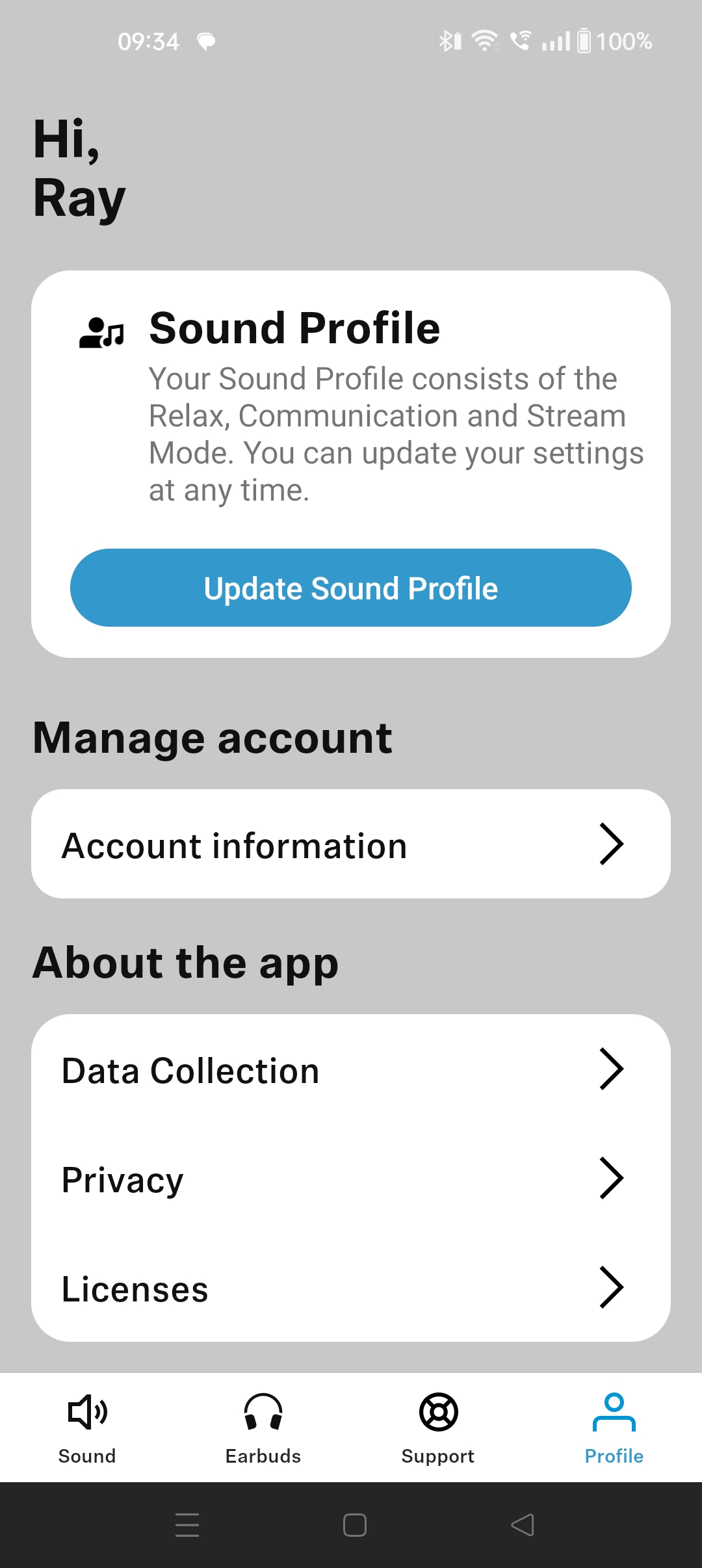This is a detailed screenshot taken from a cell phone, featuring a user interface with a gray background. In the upper right corner, white icons display the battery level, Wi-Fi, and cellular reception. The current time is displayed on the left.

Approximately three lines below the time, large and bolded black text reads "Hi, Ray." Directly beneath it, there is a prominent white rectangle. Positioned in the upper left corner of this rectangle, a black-filled circle with a rectangle below it is depicted alongside a unique music note symbol, characterized by circles at the ends of each horizontal and vertical line.

To the right of these icons, the bolded black text reads "Sound Profile." Below this heading, in lighter gray text, it states, "Your sound profile consists of the Relax, Communication, and Stream modes. You can update your settings at any time." Underneath this text, there is a blue-centered oval button labeled "Update Sound Profile."

Further down on the left, another bolded black heading reads "Manage Account." Inside a white rectangle beneath this, the text "Account Information" is present, accompanied by a right-facing arrow on the right side. Following this, another bolded black heading, "About the App," is displayed, with another white rectangle underneath listing "Data Collection," "Privacy," and "Licenses," each with a right-facing arrow.

At the bottom of the screen, a row of icons represents different features: sound, earbuds, support, and profile. The very bottom of the interface features a solid black rectangle.